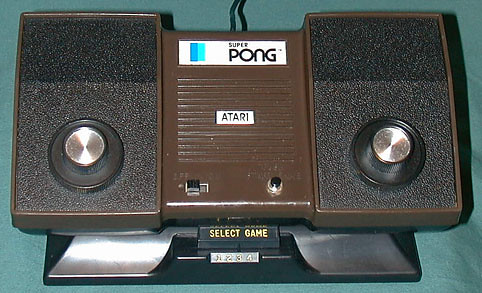A vintage photograph captures the iconic Super Pong TV controller laying on a blue tablecloth backdrop. Dominating the frame, the controller boasts its unmistakable retro design made of brown plastic, featuring dark brown film grain sections adorning both sides. The device’s centerpiece is imprinted with the "Atari" and "Super Pong" logos, with a functional switch and on button positioned at the bottom for activating the game. Flanking the main body of the controller are large, tactile twisty knobs meant for maneuvering the Pong paddles up and down on the television screen, essential for engaging in the classic game. The thick brown film grain on either side not only adds to the aesthetic but also enhances the grip of the device.

Beneath the controller, a black plastic stand labeled "Select Game" along with numbered slots 1 through 4, functions either as a charger or controller holder, suggesting practical storage and organization. The cord, serving as the device’s lifeline, stretches out from the top of the photo, trailing off into the background. Captured from a nearly head-on perspective, the photograph subtly tilts upward, providing a nostalgic glimpse into the early era of home video gaming.